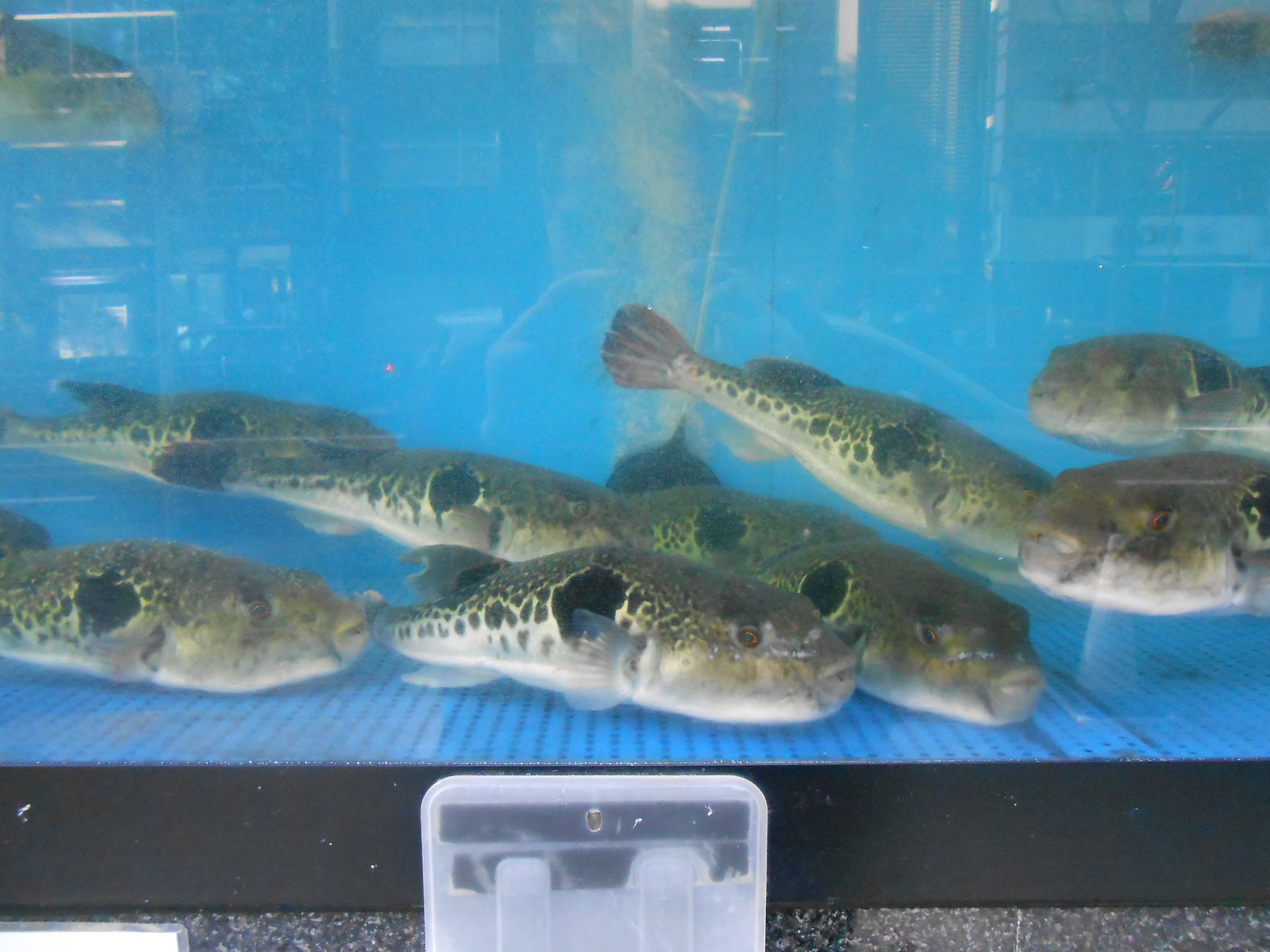This indoor color photograph provides a close-up view into an aquarium featuring a collection of puffer fish. There are eight medium-length puffer fish in total, mostly characterized by their green scales, white bellies, and large black spots on their sides. Each fish, with round faces and eyes oriented on the right, appears to be almost identical. Notably, most of the fish face towards the right, except for a couple whose heads are turned towards the camera.

The fish tank, devoid of any decorative items, has a plain blue mat at the bottom and is enclosed by a blue background. The water inside the tank is clear. A rectangular plastic container can be seen positioned at the front of the tank, and the bottom framework of the structure is composed of black steel. There is a faint reflection of the person who captured the image visible on the tank's surface.